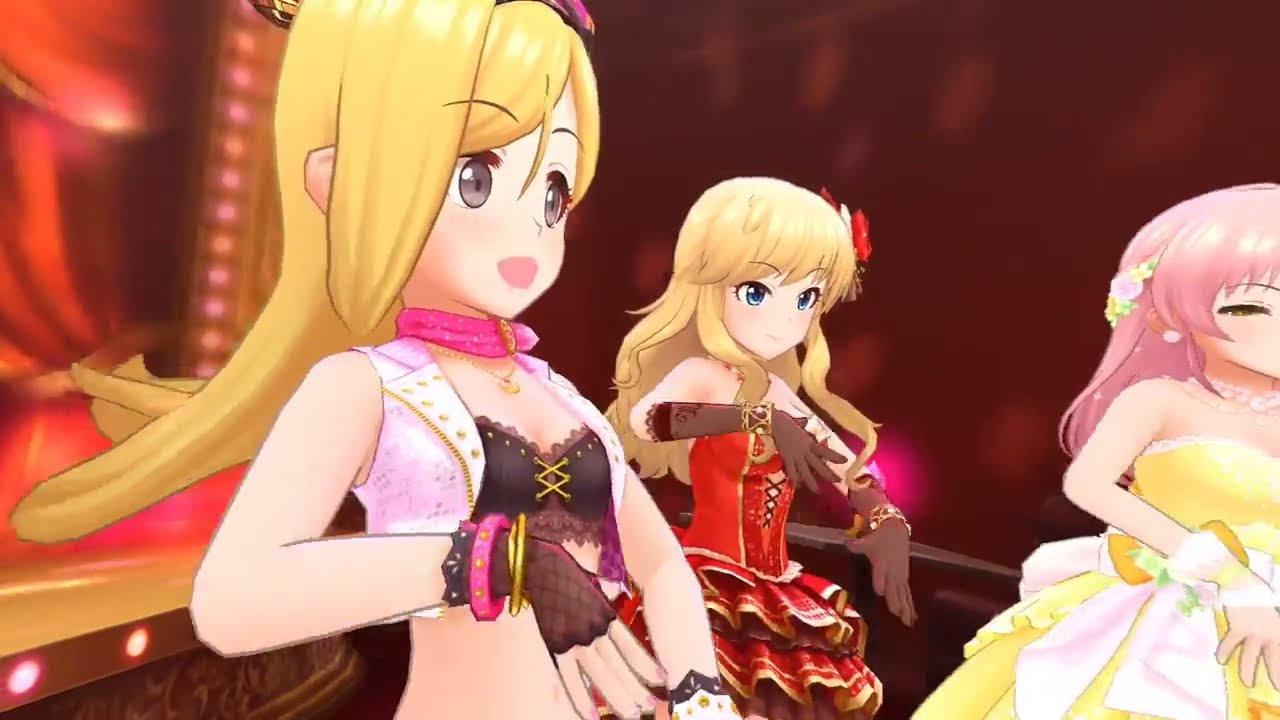In this anime-style digital artwork, three young girls with fair, peach skin are featured in elaborate and colorful outfits, set against a vibrant backdrop with yellow and red hues, suggestive of a stage or performance setting. The central figure, with long blonde hair adorned with flowers, has captivating blue eyes and is dressed in a striking red corset with a ruffled red dress. To her left stands a girl also with long blonde hair and large gray eyes, wearing a pink choker, a pink and brown top, and gold bracelets. Slightly forward in the image, she appears close to the viewer. On the right, partially cut off, is a girl with pink hair, gray eyes, and a yellow dress detailed with a white bow and ribbon, and a pink corsage on her wrist. The dynamic background, swirling with lights and dominated by warm colors, enhances the lively and festive atmosphere of the scene.